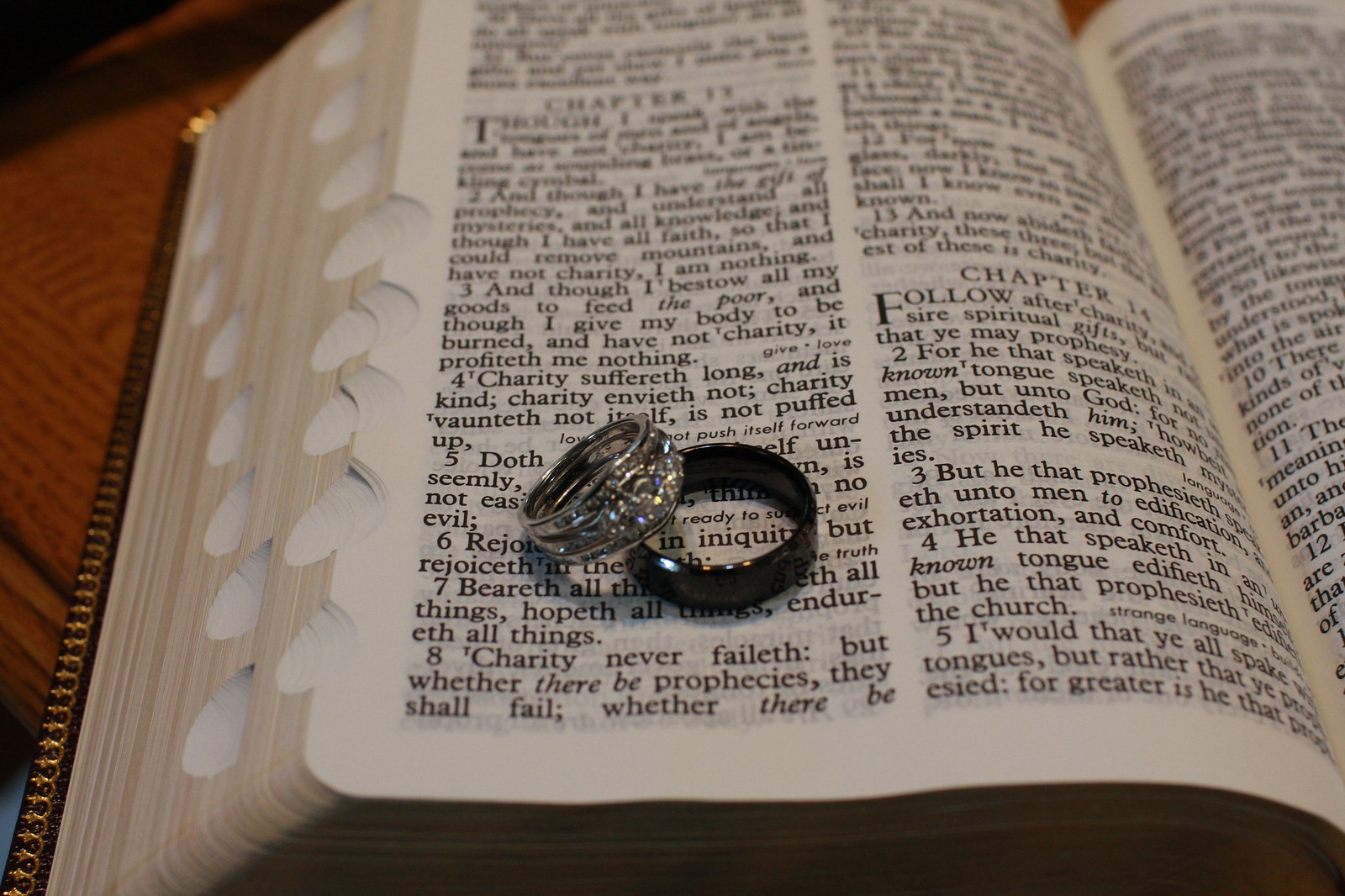This detailed color photograph captures a close-up of an open King James Version Bible resting on a wooden table, bathed in warm, dim lighting. Two rings are prominently displayed on top of the pages: a shiny white gold and diamond woman's ring, tilted and partially overlapping a larger, darker men's band. The Bible is open to chapters 13 and 14, though the specific book is not identified. The verses visible include 5, 6, and 7 of chapter 13, with verse 4 above stating, "Charity suffereth long and is kind, charity envieth not, charity vaunteth not itself, is not puffed up." This eloquent script reinforces the formal language characteristic of the King James Version. The rings, symbolizing a wedding set, delicately rest together, adding a layer of sentimental significance to the religious text below.